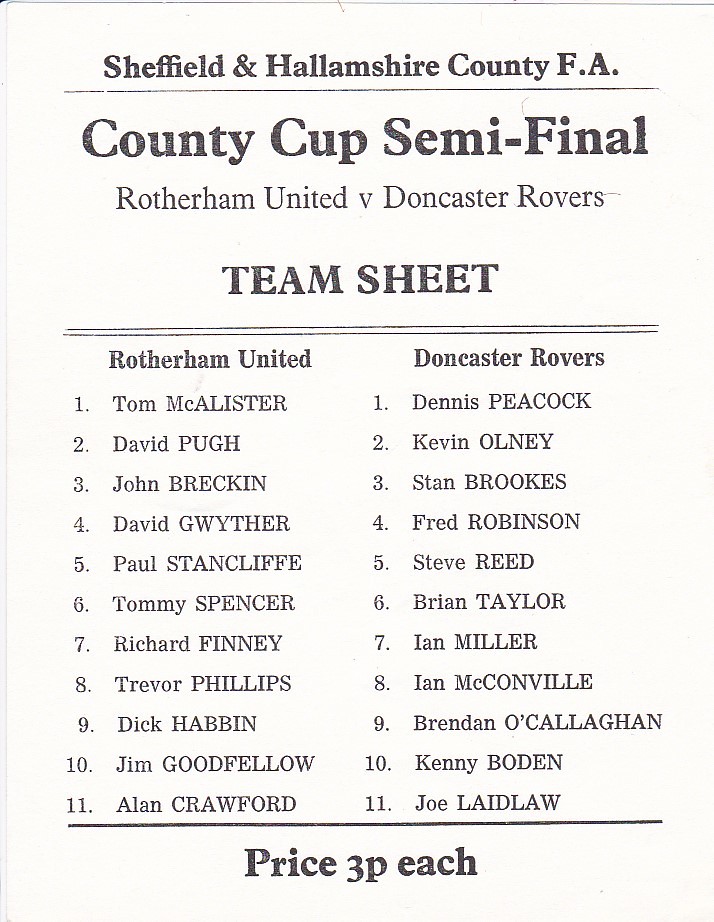The image displays a scanned team sheet from a football match, printed on a tannish yellow paper. At the top, in black font, it reads "Sheffield and Hallamshire County FA County Cup Semi-Final," followed by "Rotherham United vs. Doncaster Rovers" and "Team Sheet." Below, the roster lists 11 players for each team, with names formatted as a capitalized first letter of the first name and fully capitalized last names. For Rotherham United, the list starts with "1. Tom McAllister" and includes players such as David Pugh, John Brecken, and Alan Crawford. On the right side, the team sheet mirrors this format for Doncaster Rovers, listing their 11 players. Additionally, at the bottom, it notes the price as "3p each."